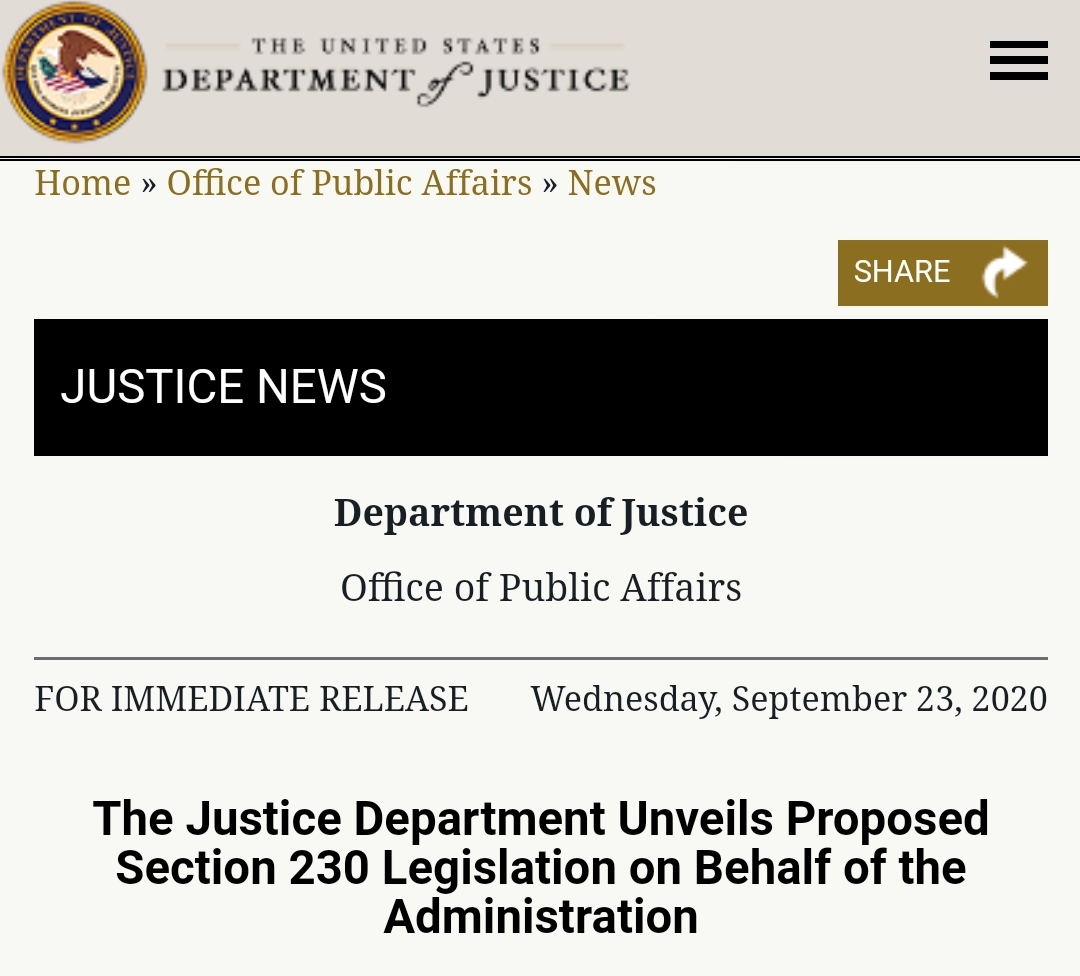The image is a screenshot from the Department of Justice website, featuring key details about a recent update. At the top of the page, the official United States Department of Justice title is prominently displayed alongside its logo to the left. To the right, there are three horizontal bars symbolizing a menu. Just below this section, the navigation options—Home, Office of Public Affairs, and News—are listed in brown font.

On the right side, there's a brown rectangular box with the word "Share" in white, accompanied by a white curved arrow pointing to the right. Below this, a black rectangle contains the text "Justice News" in white.

Further down, it mentions "Department of Justice, Office of Public Affairs," followed by a black horizontal line. Under this line, the text "For immediate release, Wednesday, September 23rd, 2020" is displayed. The title "The Justice Department unveils proposed Section 230 legislation on behalf of the administration" appears in bold black letters. This text is not hyperlinked, suggesting it is simply a headline and not clickable.

No additional information or text is included in the screenshot.